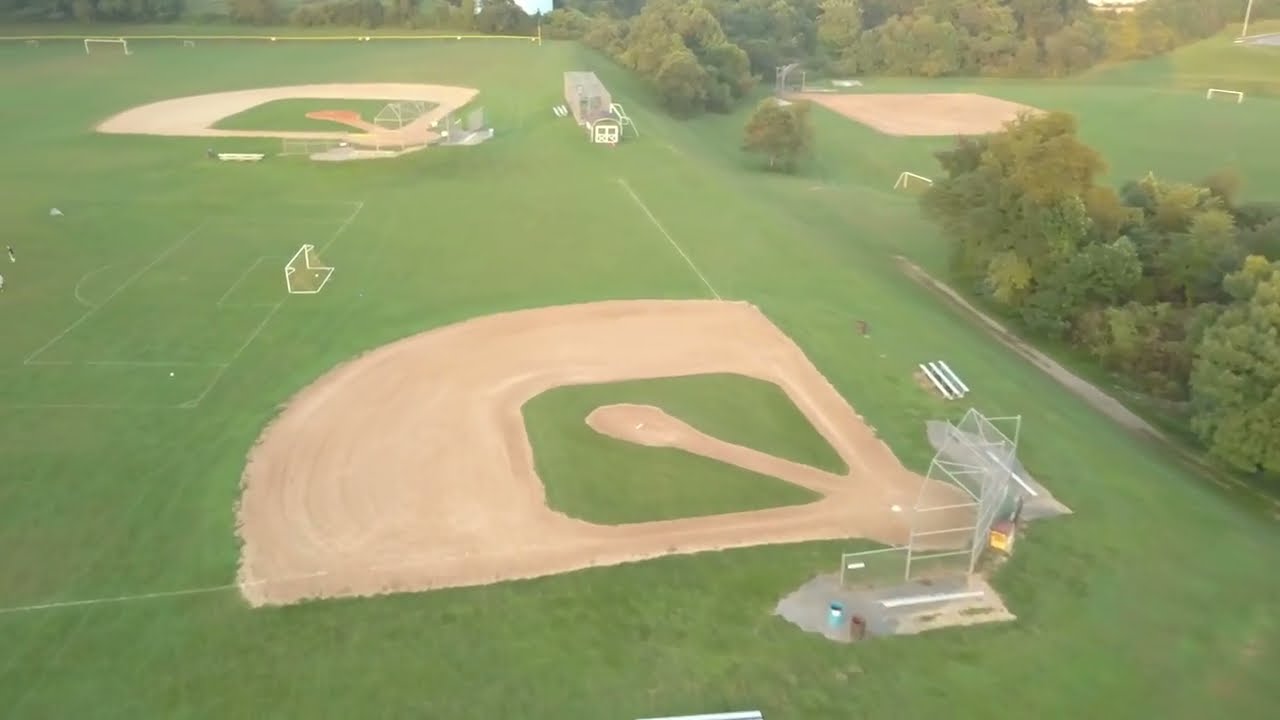The aerial image captures a sprawling recreational park predominantly designed for baseball but also accommodating soccer. Dominating the scene are three distinct baseball diamonds with signature brown dirt infields and expansive green outfields. The largest grass area features two baseball fields positioned side by side, with a small, movable white soccer goal nestled between them, intended presumably for youth soccer. To the right, there is another large grassy section hosting a third baseball diamond, accompanied by multiple soccer goals scattered around it. All three baseball fields are contained by tall, lush, bushy trees that provide a picturesque boundary to the park. A backstop, characteristic of baseball fields, is visible behind one of the diamonds. Additionally, a trailer is situated centrally, possibly for equipment or administrative purposes. The entire setup is indicative of a versatile sports park, well-suited for both baseball and soccer, and is likely a hub for community sports activities.